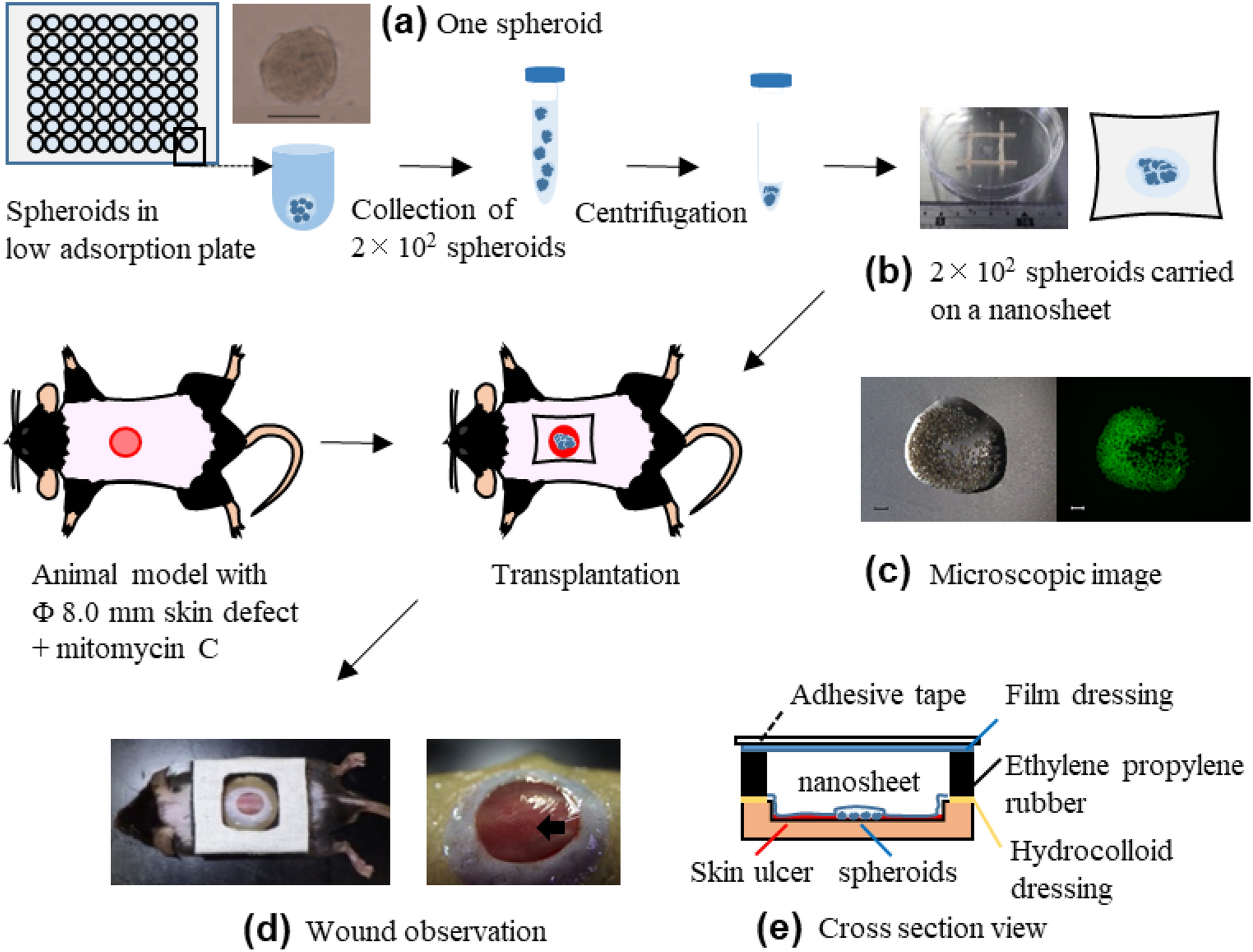This scientific diagram details the process of conducting an experiment involving mouse models, visually articulated through a series of images and diagrams labeled from A to E. 

In the top left corner, the image is labeled "spheroids in low absorption plate," showcasing a collection of circular spheroids on a grid. Adjacent to this is a depiction involving "spheroids carried on nano sheets," represented by a square with a tic-tac-toe-like grid pattern. The subsequent illustration demonstrates the centrifugation process with test tubes, highlighting how spheroids are separated.

The middle section includes a side-by-side display of spheroids under a microscope, offering a close-up view of their structure. Below these, there is a sequence related to animal models: it starts with a detailed drawing of a mouse lying flat, labeled as having an "8mm skin defect," where a section of its skin appears to be excised.

Further beneath, an additional image portrays a live mouse specimen with a noticeable circular skin defect, used to highlight the experimental procedure visually. To the right, the diagram concludes with a "cross-section view," providing a cutaway perspective of the skin defect, likely to illustrate depth and tissue involvement.

This comprehensive visual representation appears to guide the observer through each meticulous step of the experimental procedure, from handling spheroids to visualizing and documenting the effects on a mouse model.